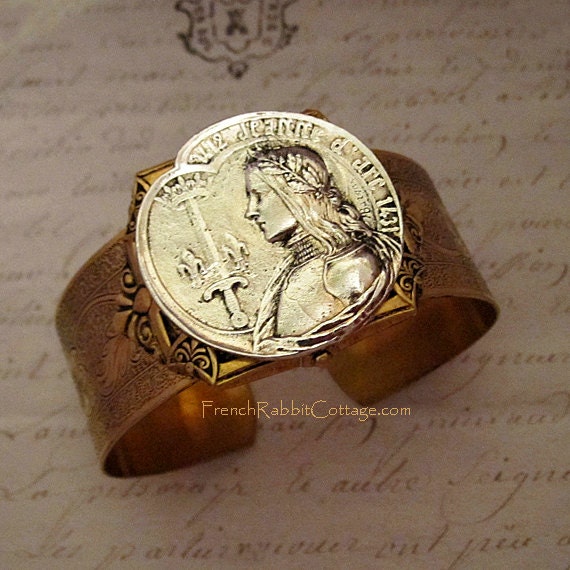This image showcases a striking historical artifact, likely a bracelet, photographed against a grainy white backdrop adorned with cursive Latin writing and an ornate crest at the top. The thick, rounded bracelet, colored in a copper-gold hue with intricate black etchings along its outer sides, features an opening at the bottom, making it a clasp design that can be adjusted to fit around the wrist. The bracelet prominently features a brilliant, traditional gold medallion at its center, engraved with a depiction of a warrior woman, likely Jeanne d'Arc, wearing a headdress or crown of thorns and holding a sword, with the year 1431 inscribed around her. Below this detailed imagery, the text ‘FrenchRabbitCottage.com’ is displayed in gold, linking the artifact to its likely website.